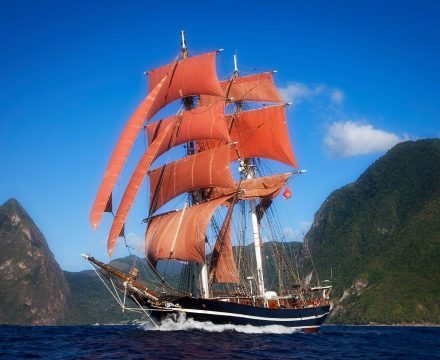This photograph, captured on a mostly square medium, showcases a large, beautifully designed sailing ship reminiscent of those from the 1800s or perhaps a bit earlier or later. The ship, likely a replica of an old wooden vessel, features two towering masts adorned with multiple unusual reddish, rust-colored sails—four rectangular sails on one mast and three on the other, along with two triangular sails at the front. It is depicted cruising through dark blue, smooth waters, with white waves breaking at its bow. Surrounding the ship are steep, rugged mountains draped in green foliage, hinting at an early summer day. The sky above is a vivid, deep blue with minimal cloud cover, growing lighter toward the horizon. Though the ship appears distant and devoid of visible crew, it commands the scene against the backdrop of lofty hills and possibly some small structures at the water's edge, emphasizing the ship as the focal point of this picturesque, serene setting.